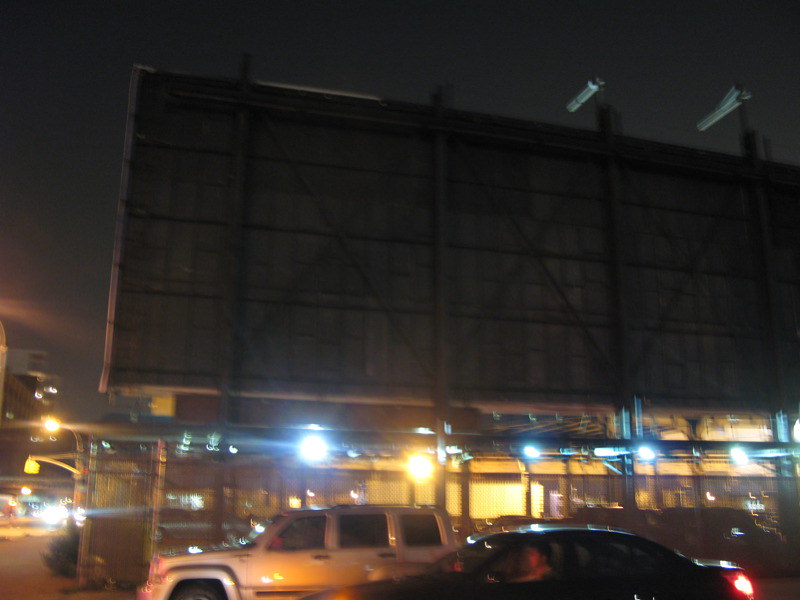This nighttime photograph captures a grainy, somewhat blurry view of an area featuring cars and a large billboard. In the foreground, you can see two vehicles—one appears to be a black sedan and the other a silver, boxy people carrier or jeep. These cars are parked side by side, facing the left side of the frame. There's a suggestion that the cars may have drivers inside, though the photo's blurriness makes it hard to confirm. Dominating the background is the back of a massive billboard, which stands tall with a complex frame of vertical, horizontal, and diagonal supports forming X shapes. No advertisements are visible on the billboard, but several mounted lights suggest its dual role for drive-in movies or daytime advertising. The pitch-black sky adds to the darkness, save for some glowing streetlights beneath the billboard, causing slight distortions in the image due to glare. Additionally, a faint cityscape can be discerned in the background amidst these conditions.